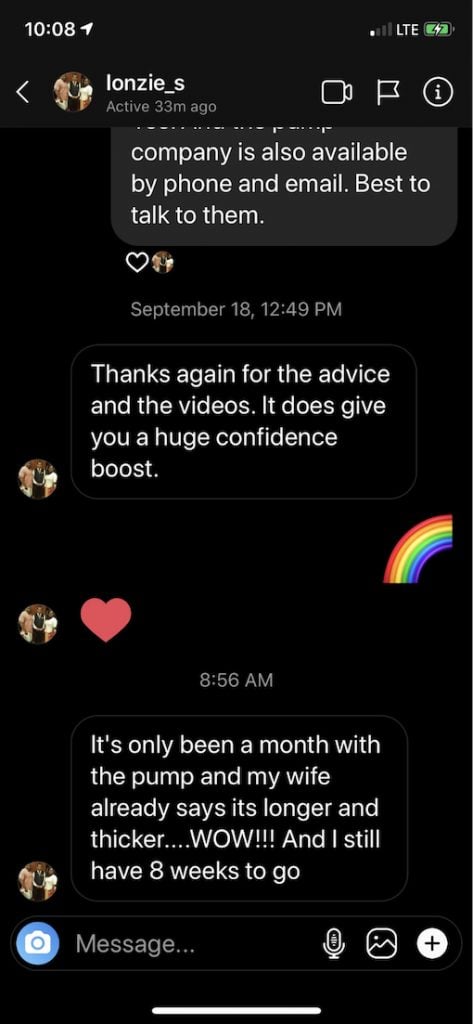The image depicts a smartphone screenshot, starting with the status bar at the top. It shows a black background with the time "10:08," a signal strength icon featuring an upward-pointing arrow and four bars (only one of which is lit up in white while the others are gray), the label "LTE," and a battery icon that appears green and contains a lightning bolt.

Below this, there’s a section with an icon of an arrow pointing left, followed by a circular avatar of people labeled "Lonzi_S," showing that they were active 33 minutes ago. To the right of this are icons of a video camera, a flag, and an eye.

Next, there is a partially visible gray speech bubble that reads, "company is also available by phone and email, best to talk to them." Underneath, there is a white-outlined heart and the same circular avatar of the people. The text "September 18th, 12:49 PM" is below this section.

Following this, on the left side, there’s another circular avatar of people next to a speech bubble that says, “thanks again for the advice and the videos, it does give you a huge confidence boost.” On the right side, there is a rainbow icon. 

Below this on the left, there is the same circular avatar of people. Next to it is a red heart icon, with the text underneath showing "8:56 AM." The next speech bubble from the same user states, “it's only been a month with the pump, and my wife already says it's longer and thicker... wow!!! and still I have eight weeks to go.”

At the bottom of the screen, there is a rectangular input area with rounded ends containing a blue circle with a camera icon on its left. The text "message..." followed by a microphone, picture, and a circle with a plus sign appears, and at the very bottom, there is a white bar.